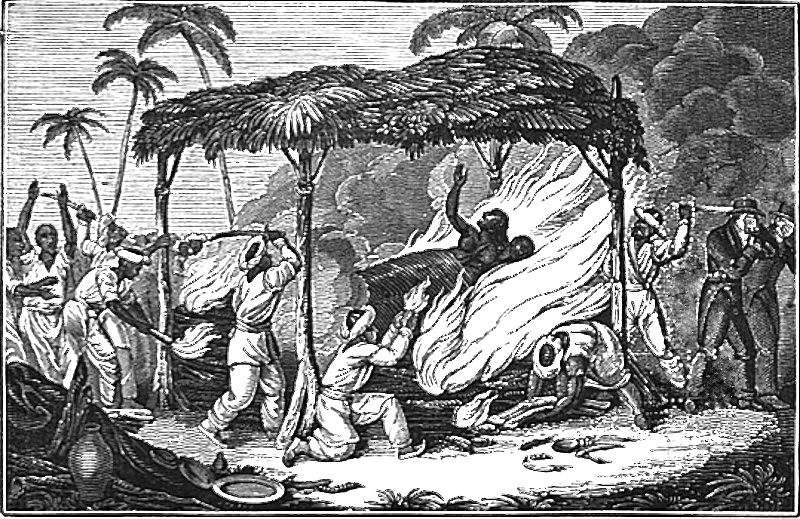This black and white etching, likely from an old book, depicts a disturbing outdoor scene. At the center, two dark-skinned individuals, perhaps bound together, lie amidst flames under a thatched canopy supported by wooden stanchions. One of them raises an arm, suggesting they might still be alive. Surrounding them are several people clad in loose white clothing, possibly servants or natives, who are actively tending to the fire. Some hold swords, hinting at a hostile action rather than a ritual. In stark contrast, to the right of the scene stand a few individuals in Western-style black suits and bowler hats, covering their faces in apparent distress or protest. The background is filled with dense black smoke and tall palm trees, while the foreground features items like jugs and plates, which could be offerings or tools.